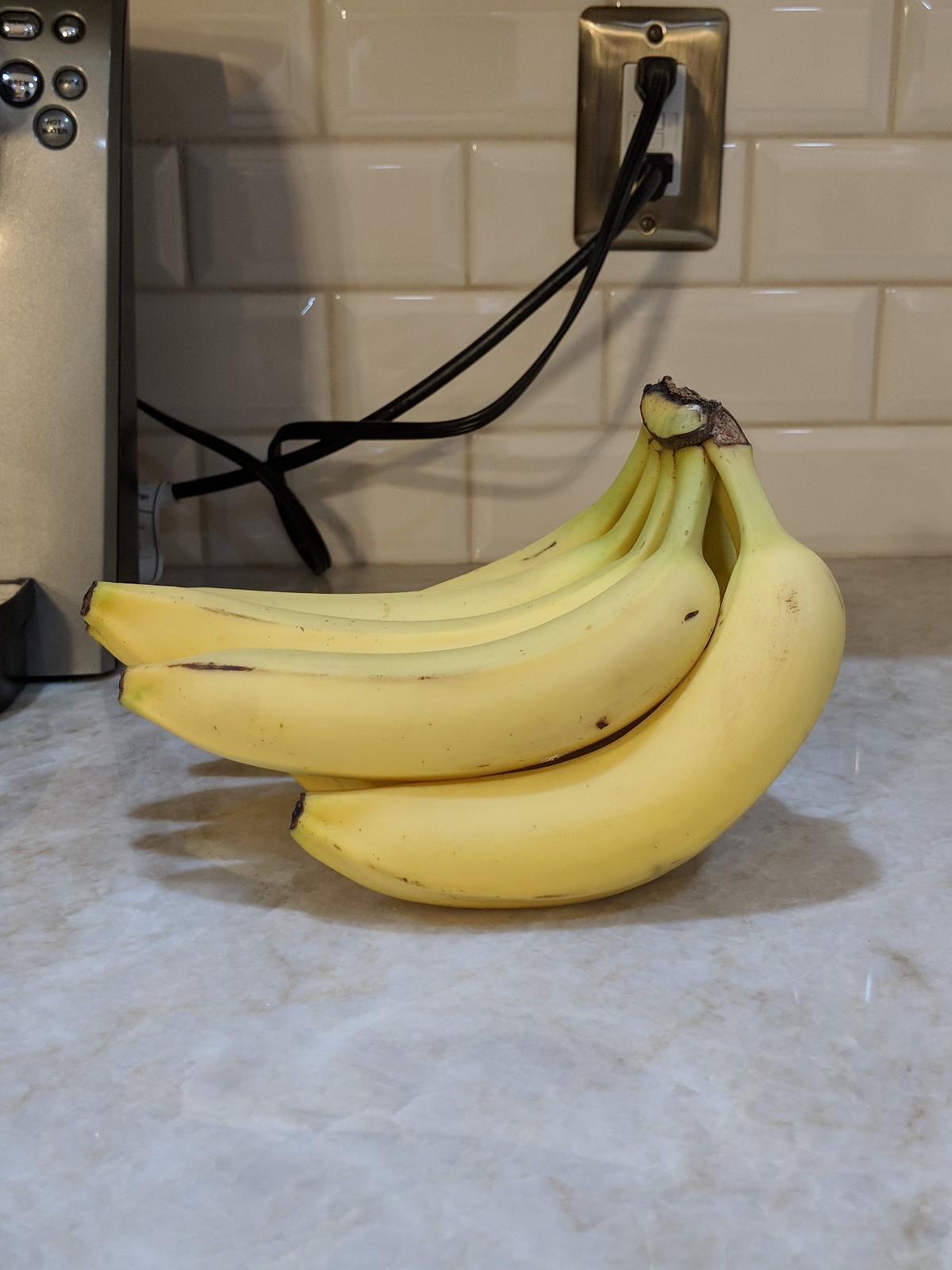The image is a vibrant, well-lit color photograph in portrait orientation, depicting a bunch of six to eight bananas resting on a gray and white marble countertop. The bananas, which are not quite ripe, form the central focus of the composition. Behind the bananas, the wall features a tan subway tile backsplash, enhancing the visual appeal of the setting. To the right on the wall, there's a metal-covered electrical receptacle with two power cords plugged in. One cord leads to a coffee maker, which is partially visible on the left edge of the image, identifiable by its five buttons. The bananas are positioned such that their stems are at the top of the photo, while their tips point toward the left, creating a balanced, everyday kitchen scene.